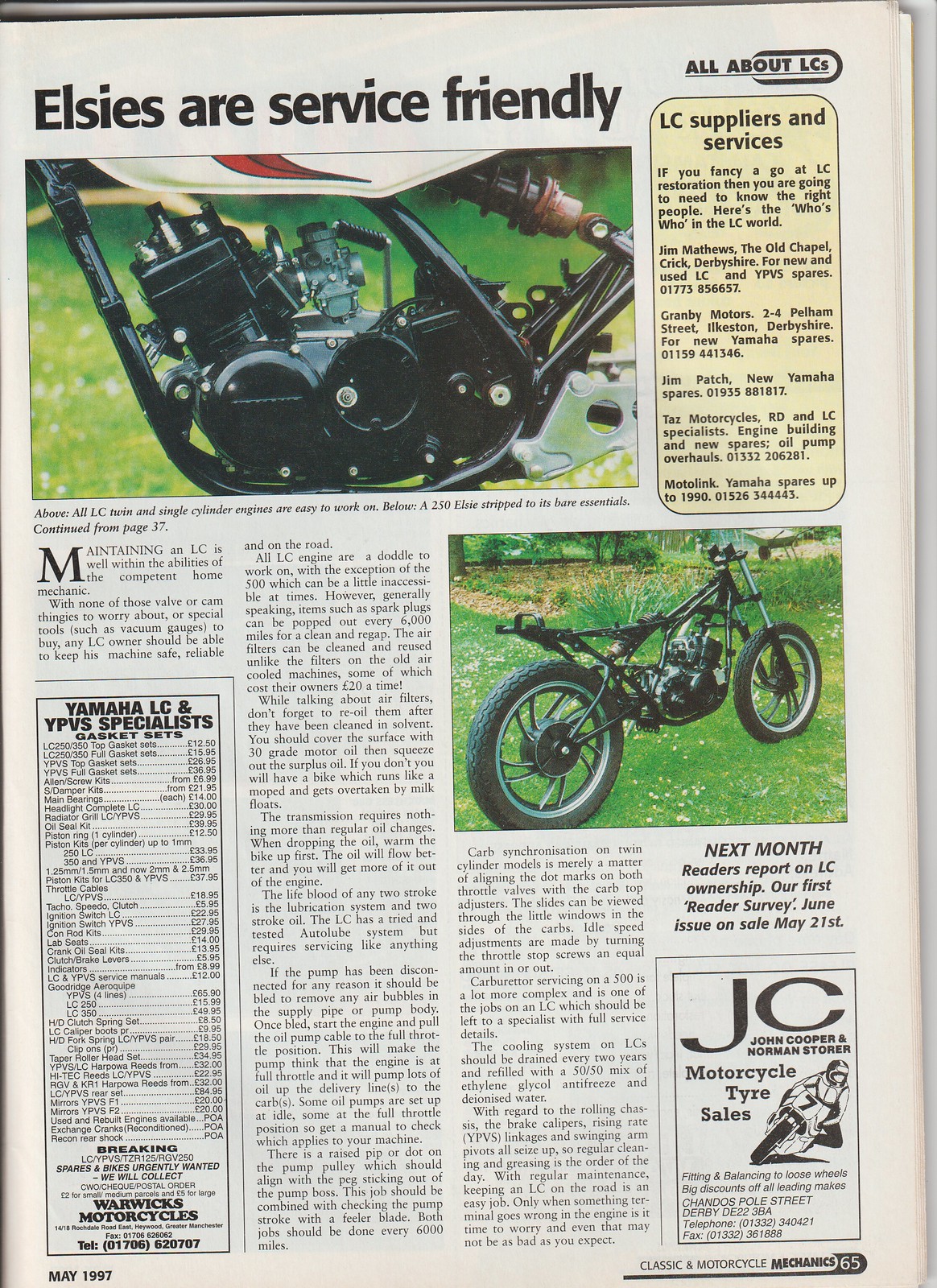This vertically aligned rectangular image appears to be a page from a magazine, indicated by the visible stack of pages along the right edge. The main title at the top of the page reads "LC's are service friendly" in large black letters. Below this title, the article features two images: the first is a close-up of a single cylinder engine on a grassy lawn, enclosed within a black border. The caption for this photo mentions that all LC twin and single cylinder engines are easy to work on. The second image, positioned further down, shows a black motorcycle or dirt bike, also on a grassy lawn, with a caption that reads, "A 250 LC stripped to its bare essentials, continued from page 37."

In the upper right corner, the page is marked with "all about LCs," while the bottom left corner indicates the magazine date as "May 1997." To the right of the main title, a light brown rectangular section with black text is titled "LC Suppliers and Services," listing several columns of information about Yamaha LC and YPVS Specialist Gasket Sets, their types, and prices. 

Additionally, an advertisement is located in the lower right corner for JC Motorcycle Tire Sales, featuring an outline of a person on a sports motorcycle and the text "JC Motorcycle Tire Sales." Further, the page previews content for the next month's issue, stating, "Next month, readers report on LC ownership," with a survey to be featured in the June issue, available for sale on May 21st.